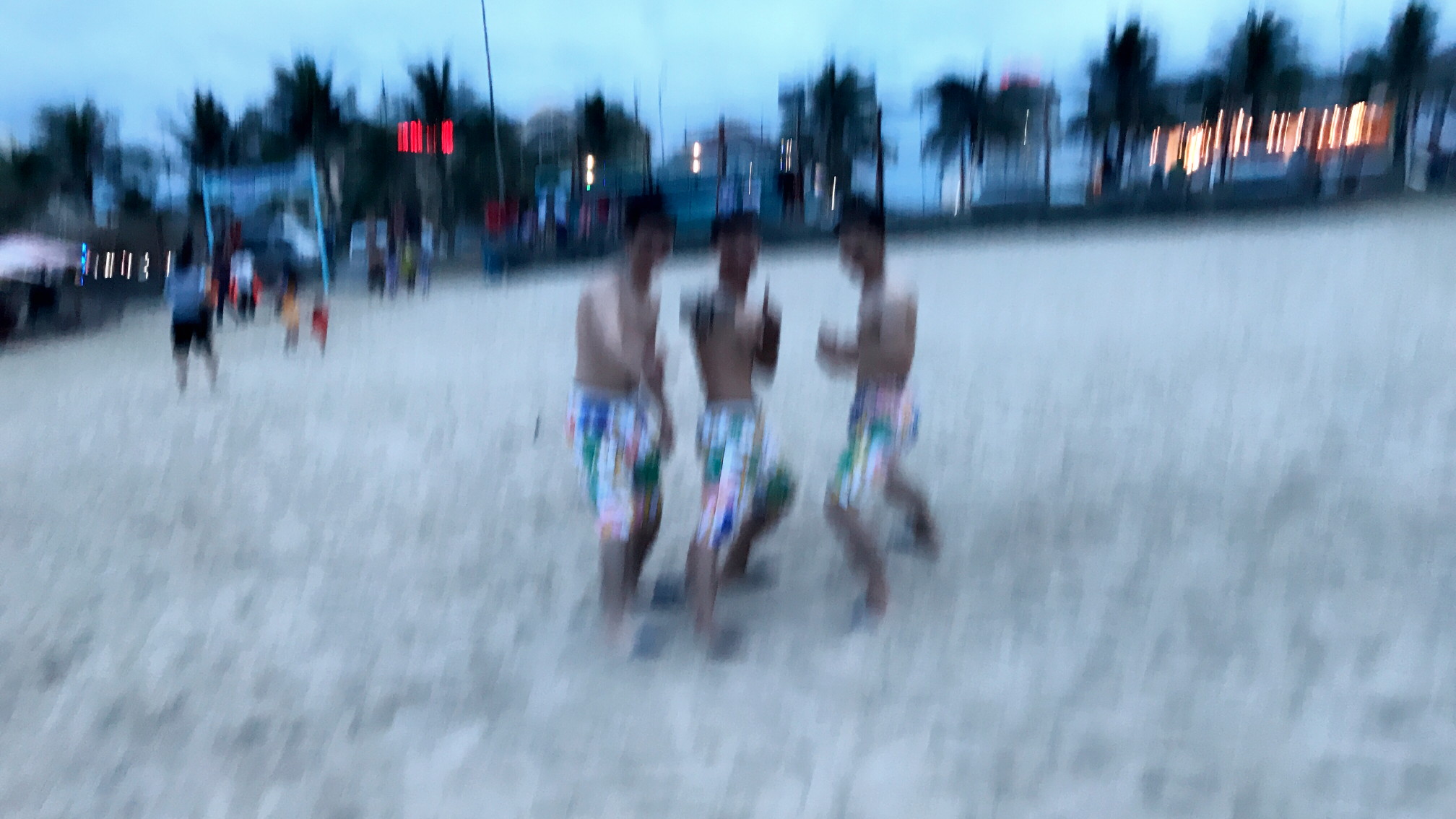The image, although out of focus, depicts three topless males with dark or black hair standing on a sandy surface, possibly a beach. They are wearing shorts, and the sand appears to have a tan or grayish hue. In the background towards the top of the image, there is a hint of greenery, possibly grass or palm trees, and some indistinct structures. Among these structures, a sign with red digital numbers or letters is faintly visible. Farther away in the upper left corner, additional people can be seen, along with two white poles that seem to support a horizontal banner or another structure with some form of writing on it.